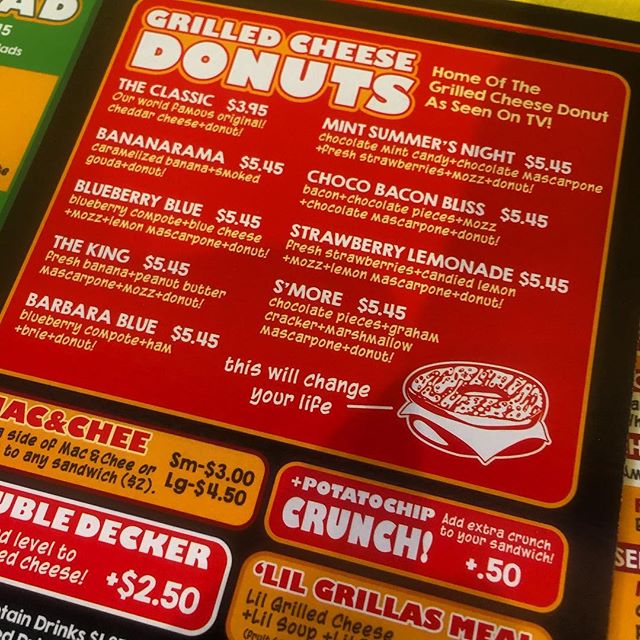This image showcases a section of a restaurant menu dedicated to grilled cheese donuts. The menu background is predominantly black, with a bold red line running horizontally across the top, bordered by black on all sides.

Prominently featured at the top of this section is a large square with a gold border and red interior, occupying nearly half the page. Within this square, the words "Grilled Cheese" appear in white letters with a bright orange border, followed by "Donuts" beneath. This section lists six different types of grilled cheese donuts, with each donut's name accompanied by its price and a brief description.

To the right of the "Grilled Cheese Donuts" title, in smaller lettering, it reads "Home of the Grilled Cheese Donut, as seen on TV." Directly below this note, four additional items are listed. There's also a playful note stating, "This will change your life," with an arrow pointing to an illustrated donut with cheese.

Further down, on the left, a small yellow rectangle with red lettering lists a mac and cheese option, including its description and price. Adjacent to this is a red rectangle titled "Potato Chip Crunch" in white lettering, suggesting an add-on that adds extra crunch to a sandwich for 50 cents.

Beneath the mac and cheese section, a red rectangle partially visible reads "Double Decker" in bold letters, with additional description and a price of $2.50. Next to this, another red rectangle at the bottom displays "Little Grilla's Meal" in bold red letters, providing details for a children's meal option.

Visible around the main section are snippets of adjacent menu sections, including a green menu with yellow details in the top left corner, and some yellow elements with lettering in the top right and bottom right corners of the image.